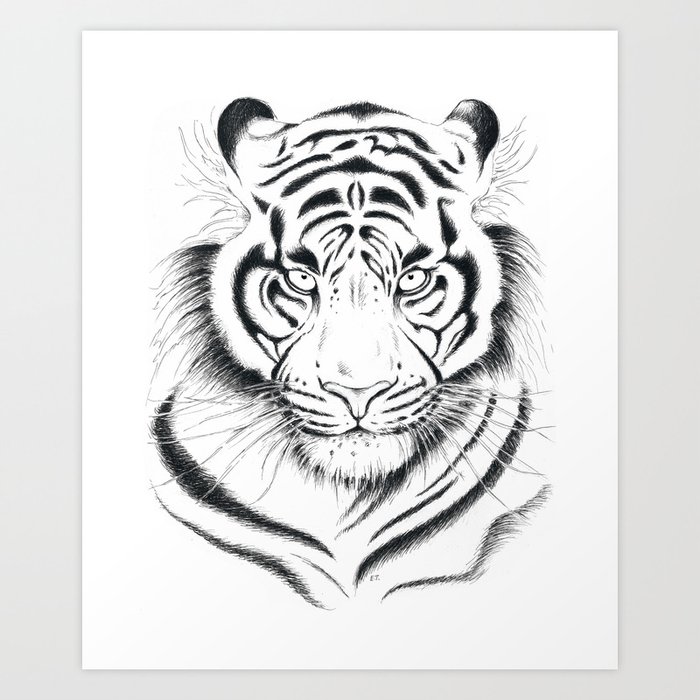This image is an intricate black and white illustration of a white tiger's face, drawn on white paper. The tiger is depicted looking directly at the viewer with symmetrical facial features. However, the stripes around its face are ornate and differ on either side. The tips of the ears are black, while the front is white. There is a distinct beard-like tuft around the tiger's chin. Whiskers and wispy lines emanate from his face, suggesting fur. The drawing includes various shades of black to highlight these details. The artist's initials are present but too small to read. The illustration, which appears to be a wall hanging, has a white background, enhancing the contrast with the tiger’s design.